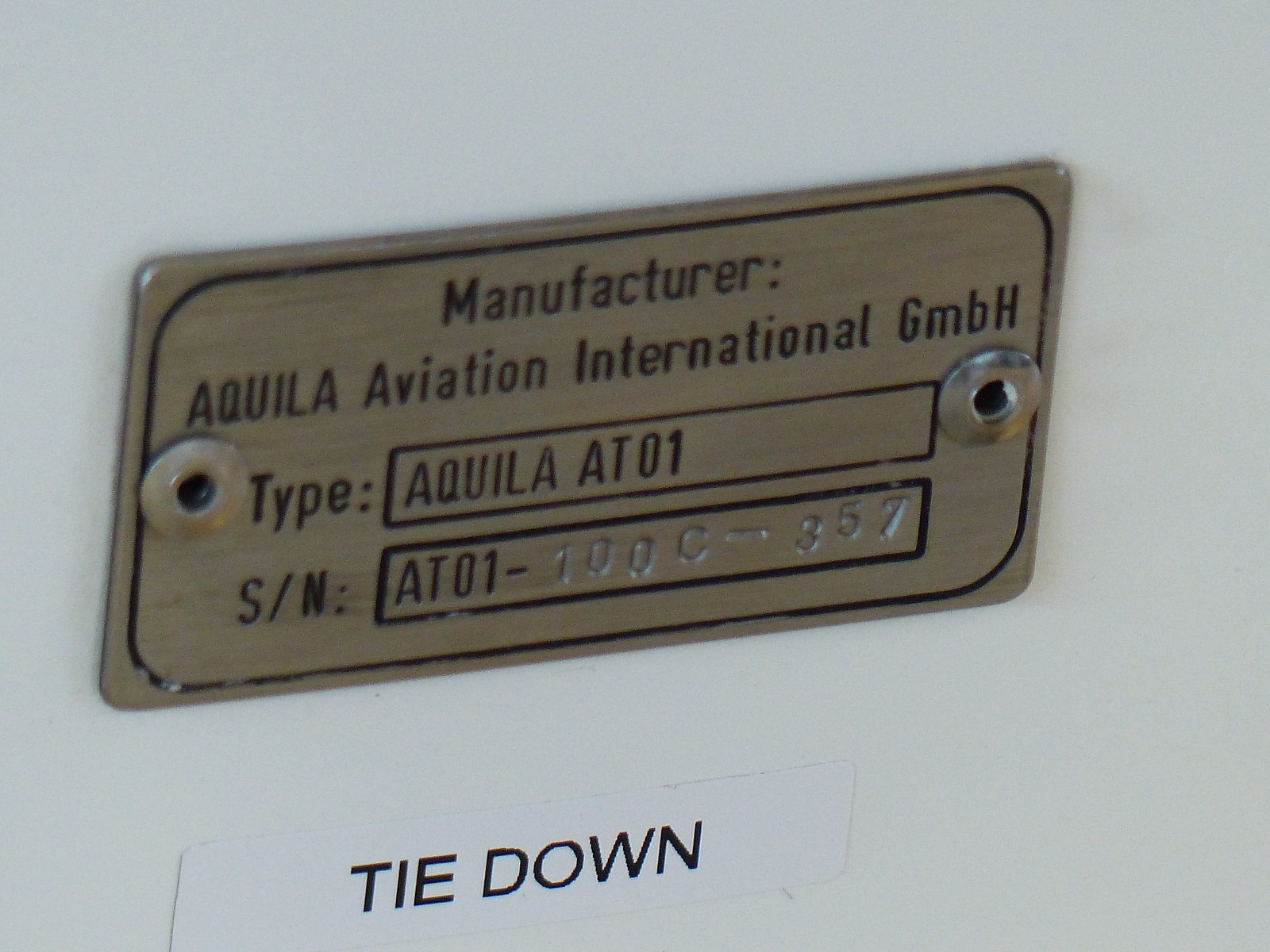The image shows a close-up of a metal label securely bolted to an unknown surface, likely related to an aircraft given the context. The background is uniformly white, providing a clean contrast to the silver-colored label. At the top of the label, the text reads "Manufacturer: Aquila Aviation International GMBH." Below this, it specifies the type as "Aquila AT01" and lists the serial number (SN) in a sequence that starts with dark lettering followed by lighter, nearly faded text, suggesting either a worn-off print or a deliberate color choice. The label also includes a small, separate plate at the bottom with the words "tie down" in black text on a white background. The entire label, including its black border, gives an impression of informative precision, possibly mounted on the side of an airplane.